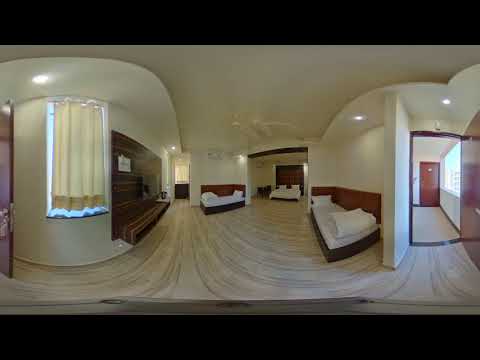The image captures the interior of a spacious room, likely a hotel suite or a large home, with multiple areas blended into one open layout. Dominating the view are several white beds adorned with white sheets and pillows, arranged in a line. The room has predominantly white walls, ceilings, and floors, with occasional black and brown accents adding contrast. The foreground includes a central area featuring two sofas, each with white pillows, contributing to the pristine look.

On the left side of the room, there's a window with a white curtain that adds a touch of softness to the scene. Adjacent to this is a brown paneled section with a mounted black TV, introducing a different texture into the space. A noteworthy feature is the doorway at the back, which leads outside through a distinct red door. This bold splash of color stands out against the otherwise monochromatic scheme. Another door, brown in color, is visible on the right side of the image, suggesting a passageway to another section of the building.

The room appears meticulously organized and spacious, enhanced by spotlights on the ceiling that illuminate the scene evenly. Interestingly, the photo has a fish-eye effect, giving the walls a slightly curved appearance that adds an unusual, eye-catching element to the otherwise straightforward composition.